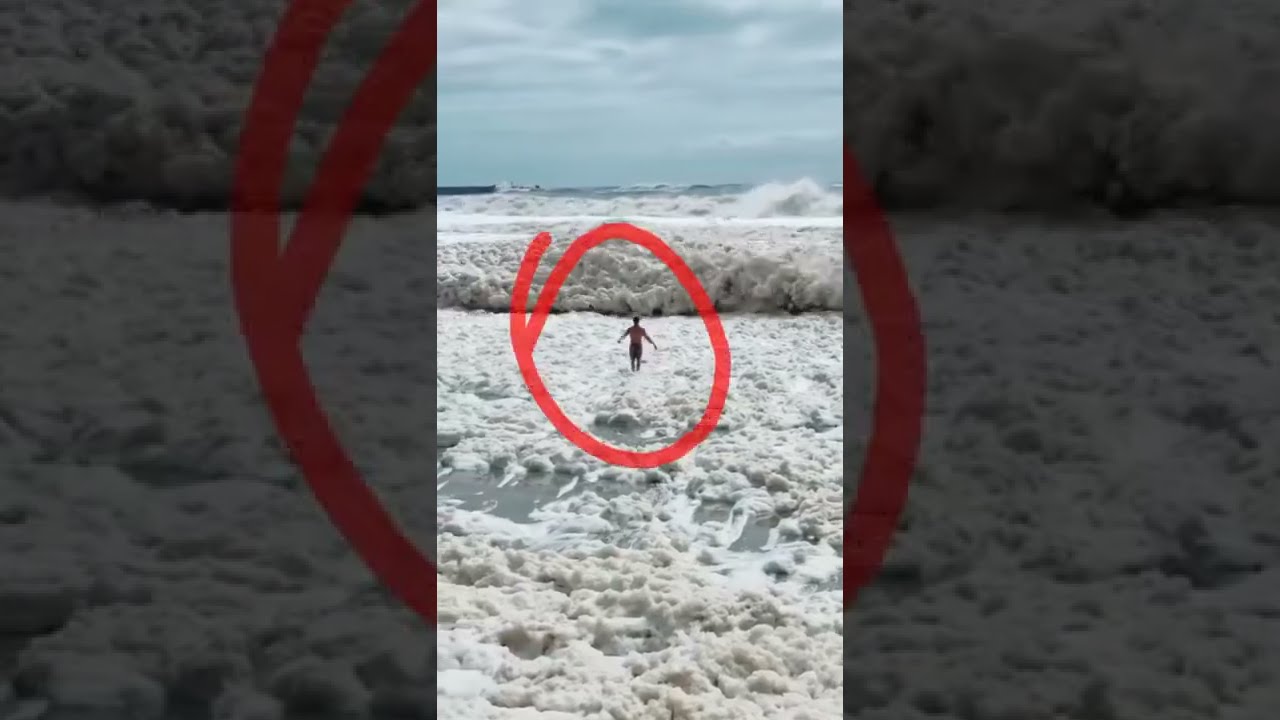The image is a rectangular photograph divided into three panels, where the central third displays the main scene. This detailed central photo shows a single figure, seemingly a man without a shirt but wearing dark pants, walking into a vast expanse of dense, white seafoam, which spans from his position far in the distance all the way to the foreground. With his arms extended, the man is captured from behind, facing away from the camera, and surrounded by white seafoam that obscures the gray sand beneath. A hastily drawn red circle highlights his presence in the middle of the photograph. The visible ocean is represented by a distant blue line on the horizon, bordered by a light gray, overcast sky. Flanking the central image, both the left and right thirds of the panel are heavily zoomed-in and darkened versions of the same photo, creating a mirrored and somewhat abstract border for the central, detailed scene.